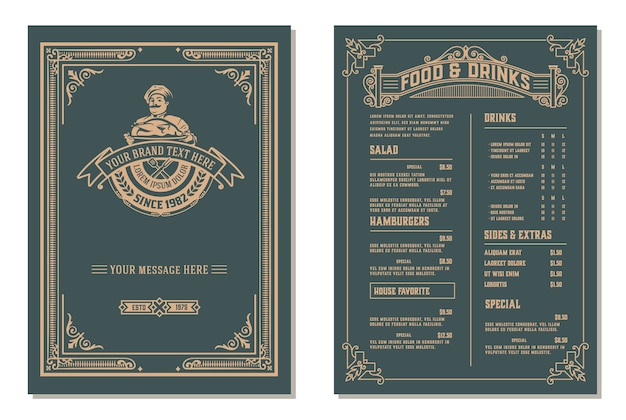The image showcases a traditional-style restaurant menu template designed with ornate stylings reminiscent of the 1800s. The menu template features two pages, front and back, displayed in a dark olive green color with beige and goldish fonts and graphics. The front page highlights a classic depiction of a stereotypical, slightly portly chef wearing a hat and mustache, holding a roasted turkey on a tray. Surrounding the chef is a decorative gold border, and a banner that reads, "Your Brand Text Here." Below the banner, there is placeholder text, "Lorem Ipsum Delore," followed by "Since 1982" and "Established 1975."

The back page of the menu is similarly styled and contains headings for different food and drink categories: Salad, Hamburgers, House Favorites, Drinks, Sides and Extras, and Specials. Under each of these categories, there is illegible sample text, serving as placeholders for actual menu items. The menu's design, with its light beige text over a deep bluish-green background, is laid out clearly and is meant to be an accessible, cost-effective option for restaurant owners seeking to create an elegant menu without extensive graphic design expenses.